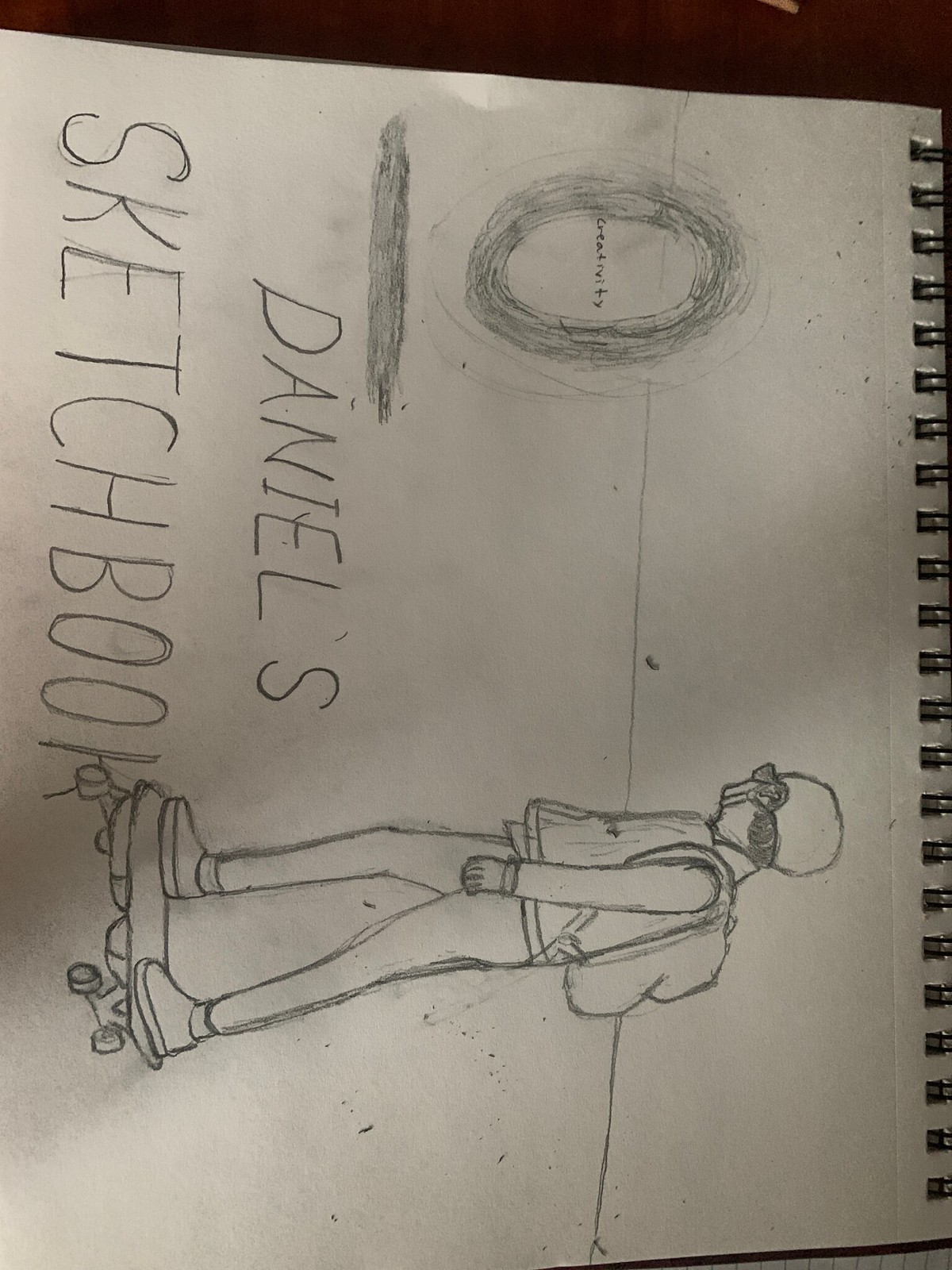This color photograph showcases an open sketchbook, prominently featuring its black spiral wire binding at the top. On the exposed page, there is a pencil drawing of a skateboarder riding towards the left. The skateboarder is detailed with safety gear, including a helmet, a jacket, pants, slip-on sneakers, and a backpack. At the bottom left corner of the page, the text "Daniel's Sketchbook" is inscribed, suggestive of ownership. Additionally, along the left edge of the page, a scribbled circle contains the word "creativity" written inside it. The sketchbook casts a noticeable shadow on the ground beneath it, indicating its three-dimensional presence in the setting. The pencil drawing, characterized by its youthful style, suggests it was created by a young artist.